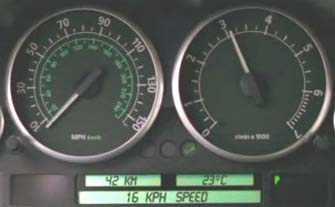The image depicts a section of a car dashboard featuring two prominent gauges. On the left is the RPM gauge, marked with silver numbers and hash marks. On the right is the speedometer, displaying speed in miles per hour with silver numbers and kilometers per hour with green numbers. Both gauges have black needles tipped in silver. Below these gauges, there's an illuminated digital display providing additional information, including the vehicle's current speed, the external temperature, and a measurement reading 42 kilometers. This snapshot offers a detailed view into the instrument cluster of the vehicle, emphasizing the dashboard's design and informative displays.